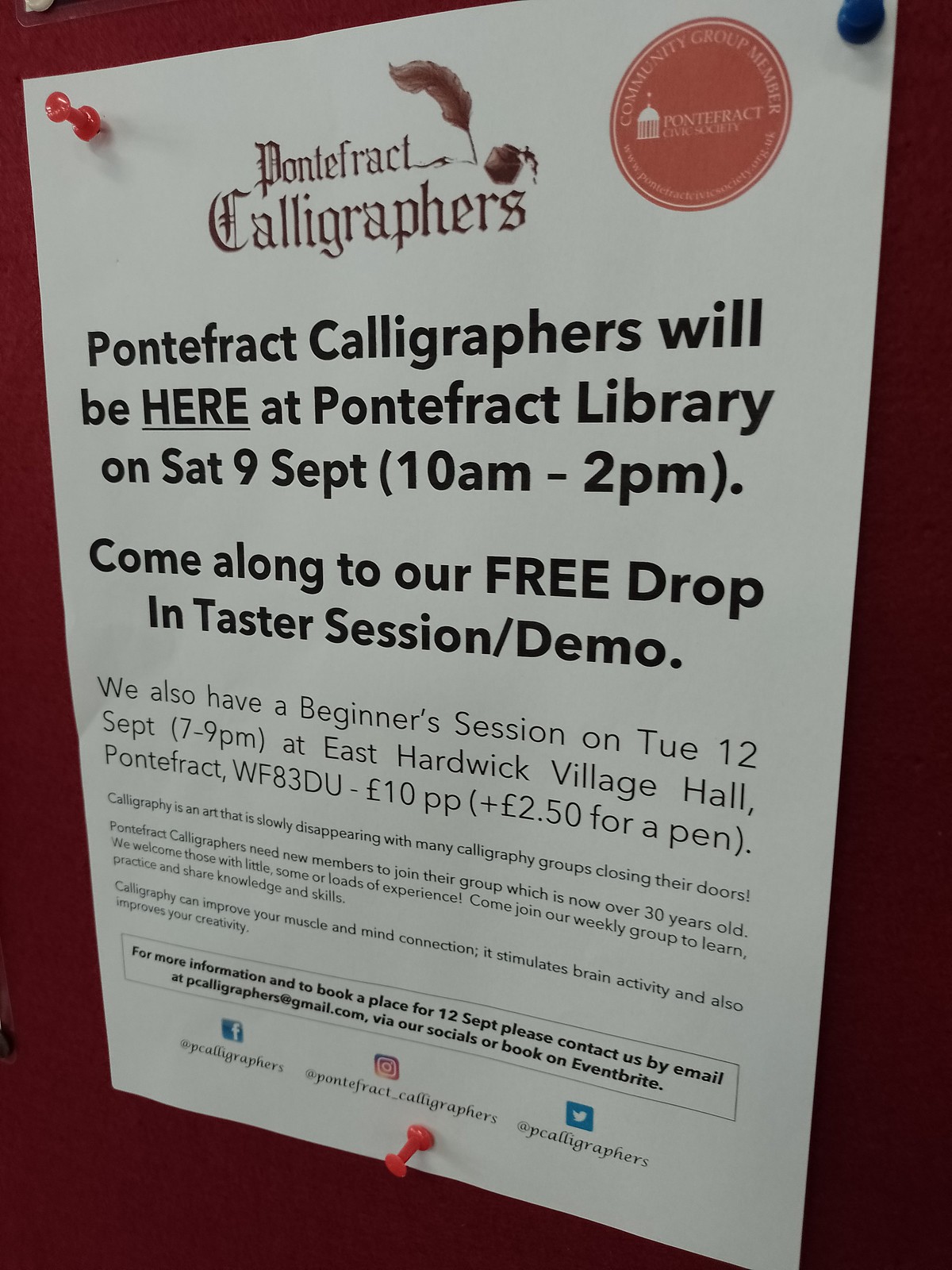The image depicts a vertical rectangular poster pinned to a dark brown chalkboard with thumbtacks—a red one at the top left, a blue one at the top right, and another red one at the bottom center. The poster, primarily white, announces an event for the Pontifract Calligraphers. At the top, "Pontifract Calligraphers" is elegantly written in cursive, accompanied by an orange symbol in the upper right corner likely representing the group. Emerging from the right of the word "Pontifract," a feather adds a decorative touch. Below, the text in black print on the white background offers detailed information: "Pontifract Calligraphers will be here at Pontifract Library on Saturday, 9 September, 10 a.m. to 2 p.m. Come along to our free drop-in taster session/demo." It continues with another event announcement: "We also have a beginner session on Tuesday, 12 September, 7 to 9 p.m. at East Hardwick Village Hall, Pontifract, WF8 3DU. £10 pp plus £2.50 for a pen." Smaller text at the bottom expands on the value of joining the group, stressing its over 30-year history and the benefits of calligraphy, such as improving muscle and mind connection, stimulating brain activity, and fostering creativity. For more details and to book a place for the 12 September session, it directs to contact via email at PCalligraphers@gmail.com or through their social media platforms on Facebook, Instagram, and Twitter (@Pontifract_Calligraphers and @P_Calligraphers, respectively). Despite some text at the very bottom being too small to read, the poster provides sufficient details for interested individuals.